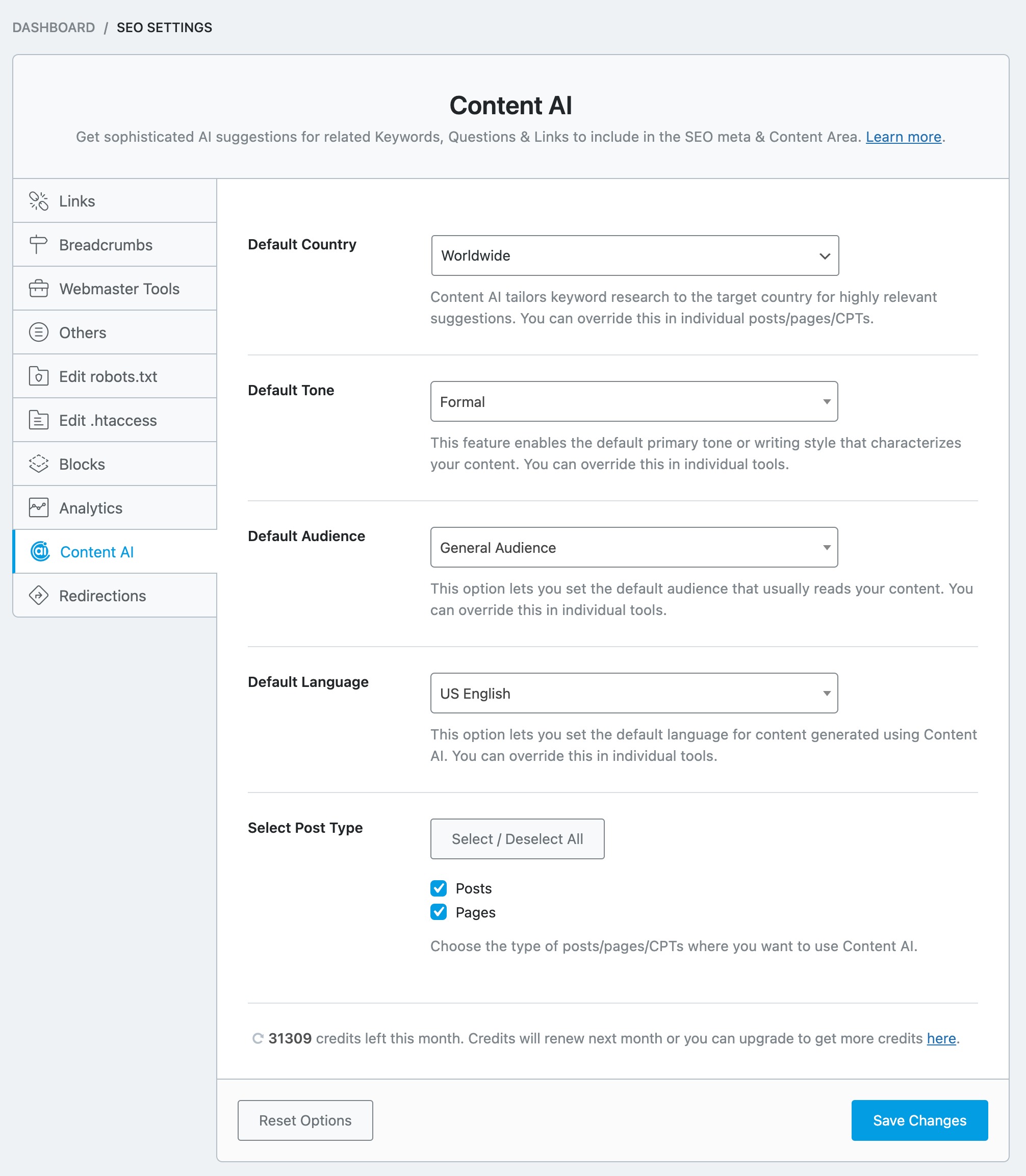This image is a screenshot of a web page from a dashboard under the 'SEO Settings' section. The background features a light gray color, whereas the main content area contrasts with a white foreground. Prominently displayed in the top middle of the page is the header 'Content AI', with 'AI' capitalized. Below the header, a descriptive text reads: "Get sophisticated AI suggestions for related keywords, questions, and links to include in the SEO meta and content area." Following this message, a 'Learn More' link is highlighted in blue and underlined.

On the left side of the page, a vertical menu lists various sections, each accompanied by an icon. The sections include:

- Links
- Breadcrumbs
- Webmaster Tools
- Others
- Edit robots.txt
- Edit .htaccess
- Blocks
- Analytics
- Content AI (currently selected and highlighted in blue)
- Redirections

Within the 'Content AI' section, several default settings are displayed:
- Default Country: Worldwide
- Default Tone: Formal
- Default Audience: General Audience
- Default Language: US English
- Select Post Type: Options to select/deselect all

At the bottom of the 'Content AI' settings, there is a 'Save Changes' button for users to apply any modifications made. 

Overall, the screenshot offers a detailed look at the 'Content AI' feature within an SEO settings dashboard, along with its customizable options and user interface design.